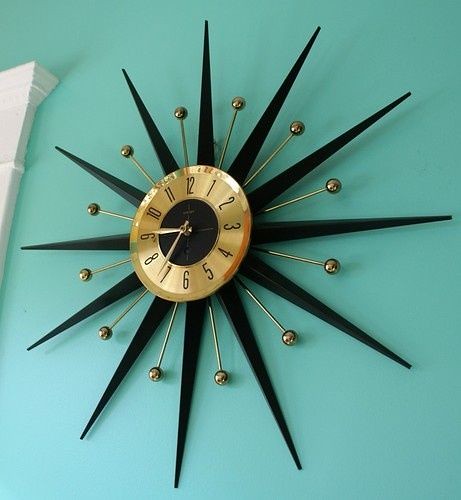This image features a large, vintage mid-century decorative wall clock, prominently mounted on a bright teal, almost Tiffany blue wall. The clock is designed in a striking sunburst pattern, with long black spikes radiating outward, each spike raised and angled to a sharp point. Interspersed between these spikes are slender gold rods, each capped with a polished gold ball, alternating all the way around the clock. The clock's face, a gold disc with a black center, displays large, black numerals and sleek, gold minute and hour hands, set to a time of approximately 8:37. A highly polished finish especially accentuates the gold detailing around the clock’s edge. The wall and clock cast a visible shadow adding depth to the scene. To the upper left side of the image, the carved frame of a doorway or window, painted white, just comes into view, adding a touch of architectural detail to the composition.